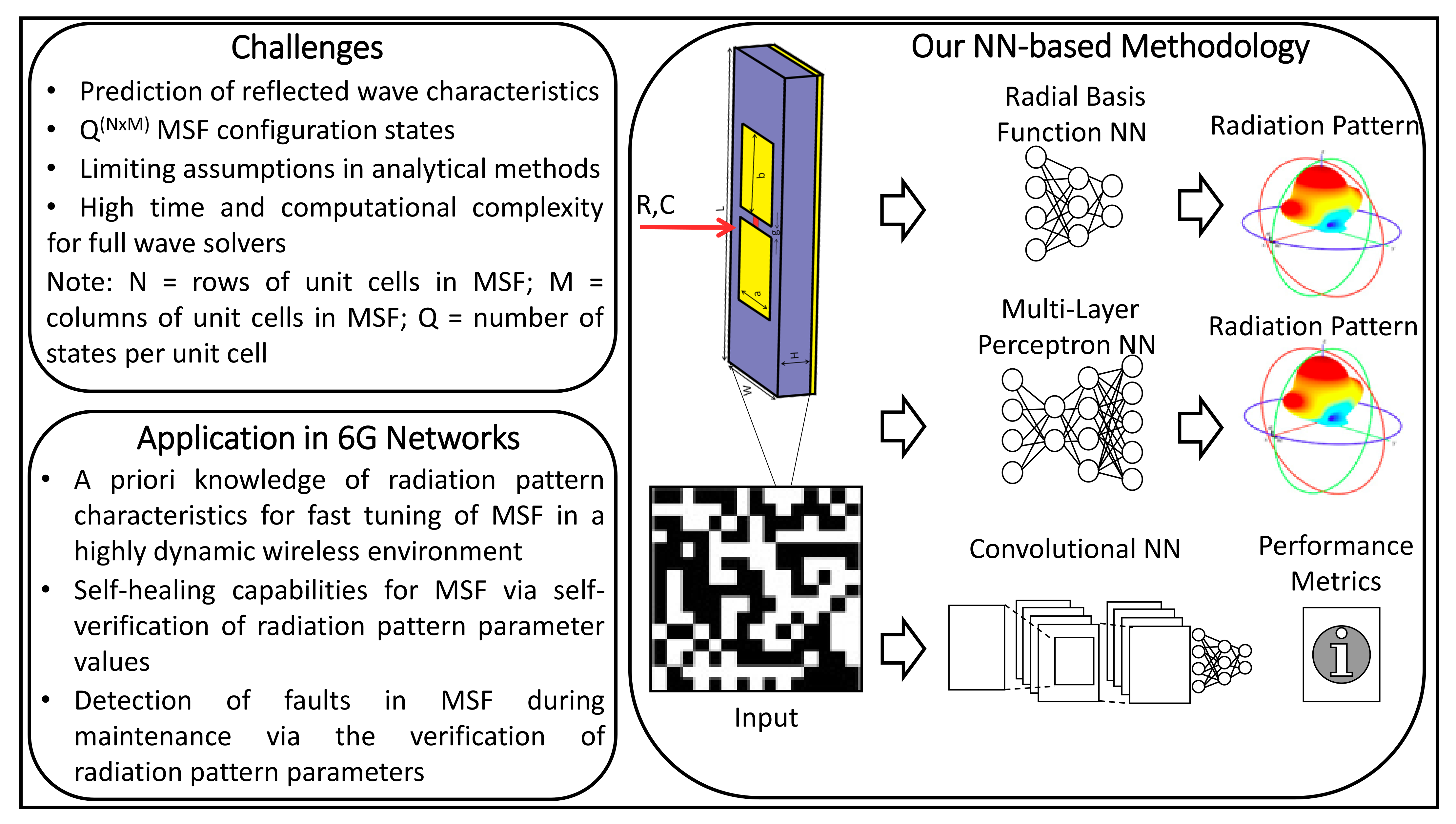This image appears to be a page from a science textbook or a PowerPoint presentation focused on the application of an RNN-based methodology in 6G networks. The primary focal points are highlighted within four rounded rectangular sections titled "Challenges," "RNN-Based Methodology," "Application in 6G Networks," and "Radiation Pattern." The "Challenges" section lists specific issues such as the prediction of reflective wave characteristics, MSF configuration states, limiting assumptions and analytical methods, and the high computational complexity of full wave solvers. The "Application in 6G Networks" discusses utilizing prior knowledge of radiation pattern characteristics to enable fast tuning of MSF in a dynamic wireless environment. On the right side of the page, colorful diagrams are used to illustrate the RNN-based methodology, RC (Radial Basis Function), and the radiation pattern, resembling a nucleus with shades of red, yellow, and blue. The detailed and intricate scientific diagrams provide a visual representation of how these methodologies are applied in advanced wireless communication systems.